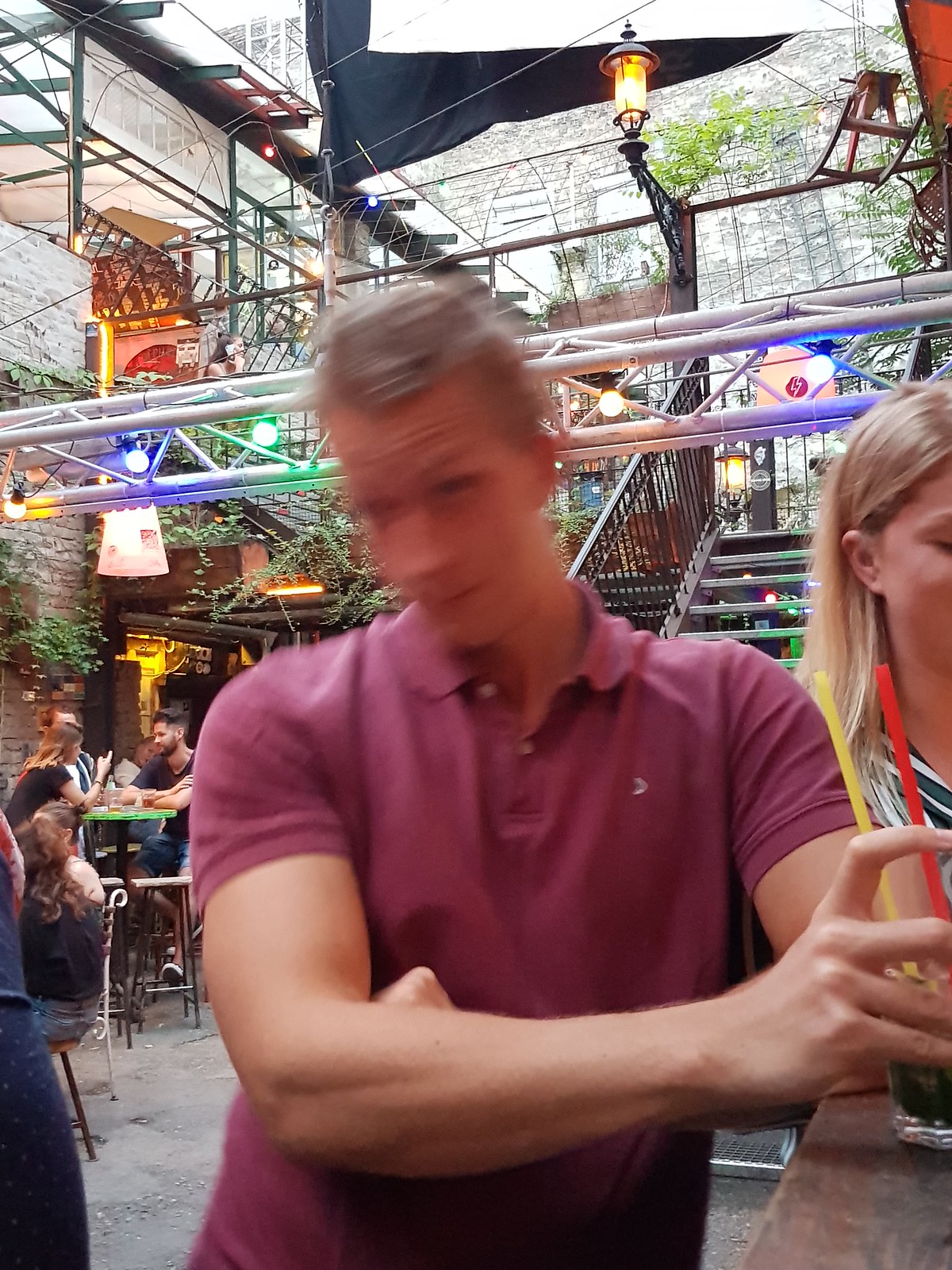This photograph, taken indoors at a bustling restaurant, features a young man in his 20s front and center, wearing a maroon, short-sleeved, collared shirt. His hair is light brown, and though his face is blurred due to movement, he is holding a drink in his right hand that has both a red and a yellow straw in it. His left arm is leaning on a counter. To his right, a young blonde woman with long, straight hair and wearing a black and white striped blouse is partially visible. In the background, there is a staircase with silver piping and a streetlight-like fixture above it. The seating area below consists of tables and chairs where several people are dining. The setting is rich with greenery, including hanging plants and baskets. The brick floor, brick walls, and abundant natural light streaming from skylights above add to the ambiance, alongside some decorative black sailcloths and various lighting fixtures.